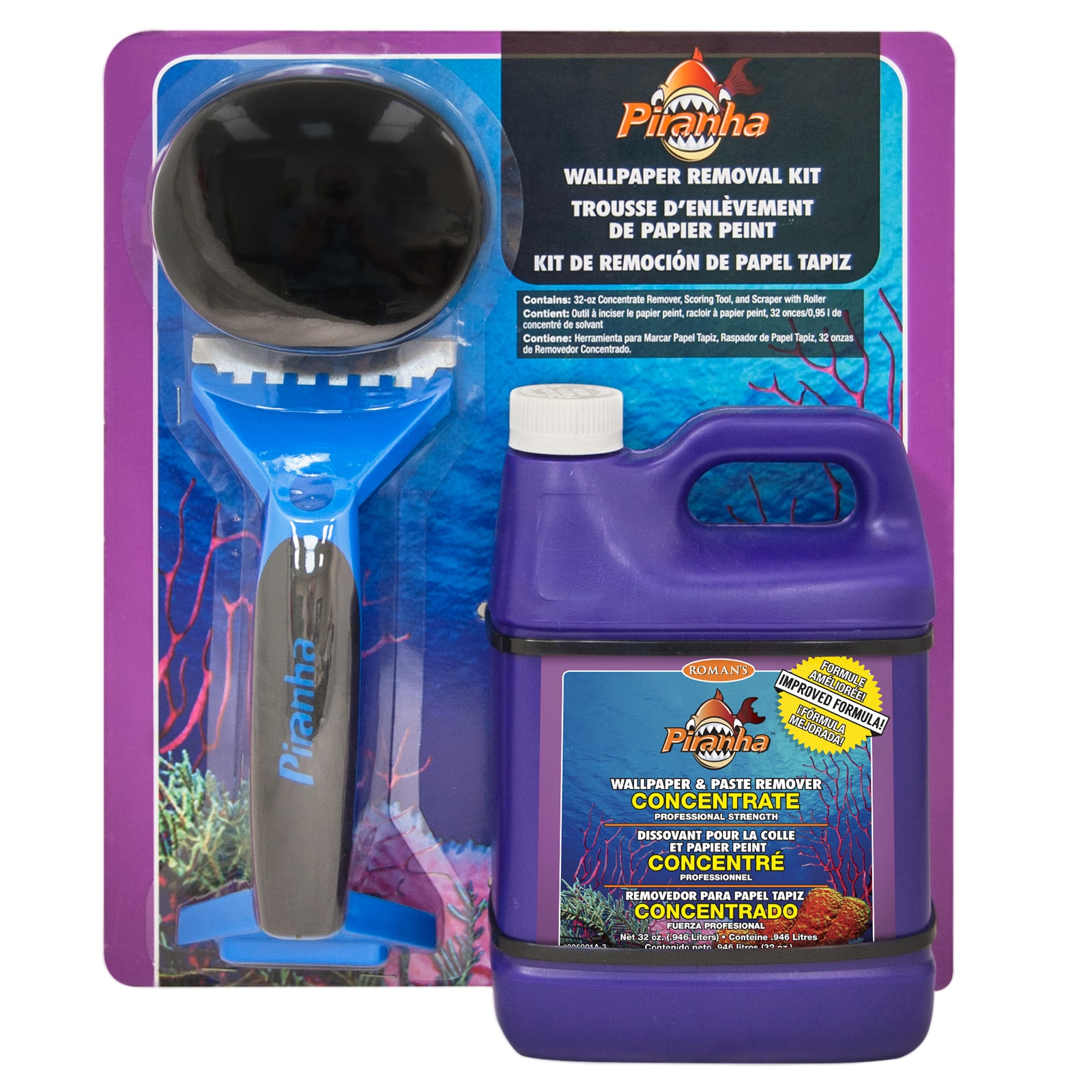The image depicts a wallpaper removal kit set against a blue ocean-themed background with a purple border. Dominantly visible on the top right is a black box featuring a red, open-mouthed piranha logo with the brand name "Piranha" written in orange letters across the fish. Below it, in white text, "Wallpaper Removal Kit" is stated along with its French and Spanish translations. The kit includes a 32-ounce concentrate remover, a scoring tool, and a scraper with a roller. Featured prominently is a purple container labeled "Wallpaper and Paste Remover Concentrate" in both English and French, with a white cap. To the left of the container is a black circular scoring tool. Adjacent to it is a blue and black scraper tool with a blue handle and a metal flat head, resembling a shovel. The word "Piranha" is written in blue vertically on its black handle. The kit components and descriptive texts are clearly detailed, enhancing the product's presentation.